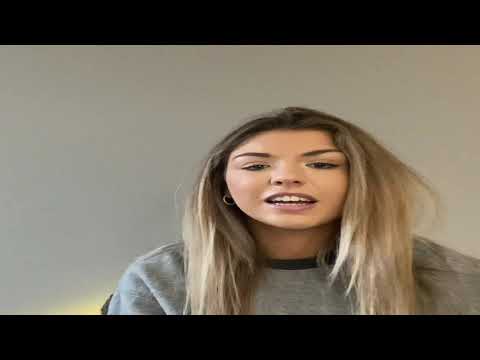The image is a close-up, high-definition photograph of a young woman who appears to be in her late teens or early twenties. She is positioned centrally, looking directly at the camera, and appears to be speaking or mid-sentence with her mouth open, revealing her teeth in a slight smile. She has long hair that is predominantly dirty blonde, with brownish roots and lighter blonde tips, flowing past her shoulders. Her complexion suggests she might be Asian, Hispanic, or of mixed ethnicity. She has tan skin and is wearing small gold hoop earrings in her right ear. She is dressed in a grey crewneck sweatshirt with a black shirt underneath, which might be mistaken for a workout sweater. The background is a plain beige wall, devoid of any other objects or people, suggesting a simple and uncluttered setting. The photo is formatted in a widescreen, television-like aspect ratio, with black borders at the top and bottom, hinting that it might be a still from a video chat or online session.